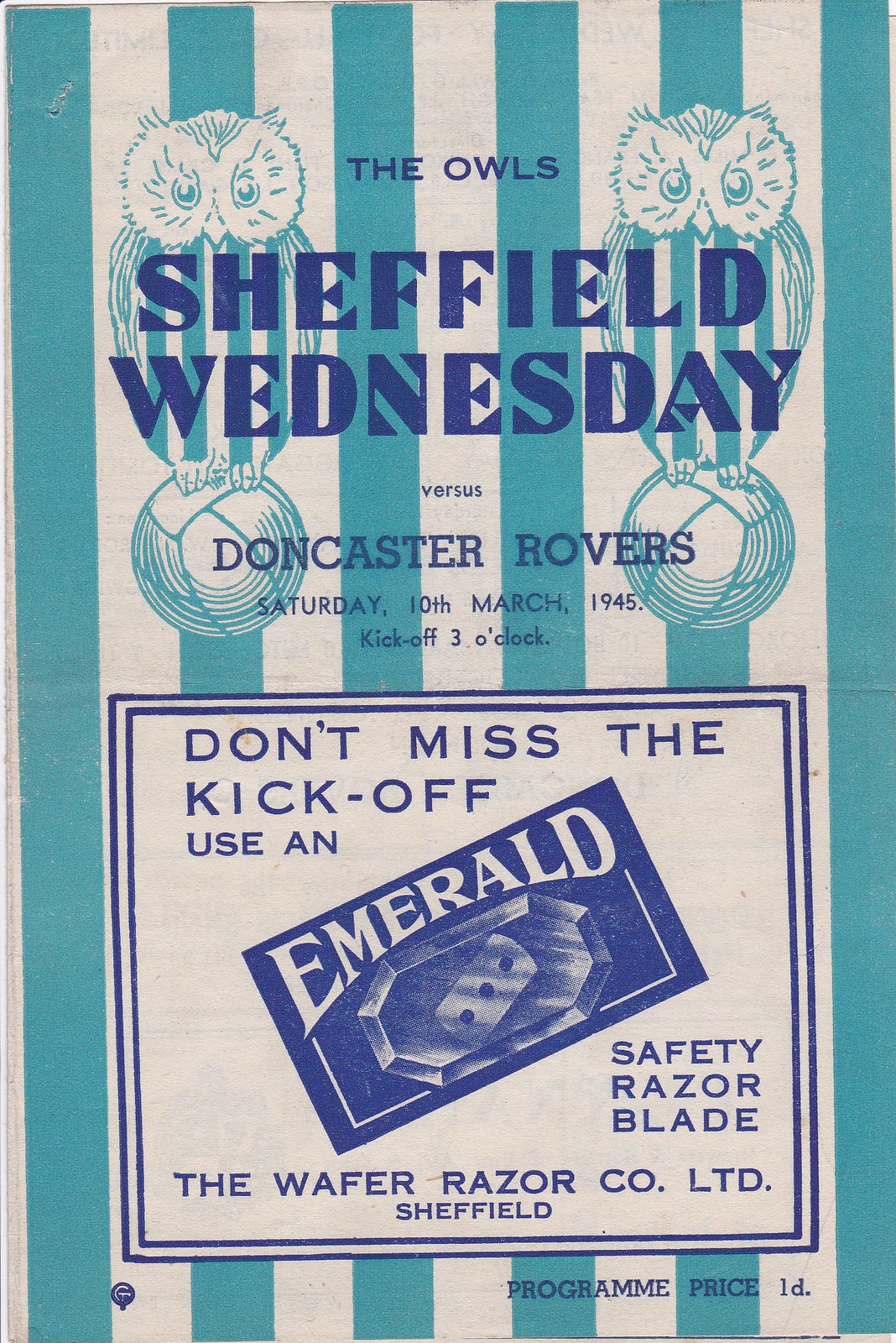The program cover features an aqua and cream color scheme with vertical stripes running up and down the page. Superimposed on these stripes are two owls; placed on the left and right sides. Between the owls, in small uppercase dark blue print, it reads "the owls." In all uppercase letters, "SHEFFIELD" is prominently displayed across the top of the owls. Below that, it says "Wednesday" followed by "versus" in smaller print, and then "Doncaster Rovers."

The owls are perched on white soccer balls, which also feature the blue and cream stripes. Detailed below this, in smaller print, reads "Saturday, 10th March, 1945. Kickoff at 3 p.m." At the bottom of the cover, there's a thin blue-outlined rectangle containing the text "Don't miss a kickoff, use a..." followed by a logo for Emerald Safety Razor. Adjacent to this logo, it says "Rafer Razor Company, Limited, Sheffield." Finally, in the bottom right-hand corner, it specifies "Program Price 1D."